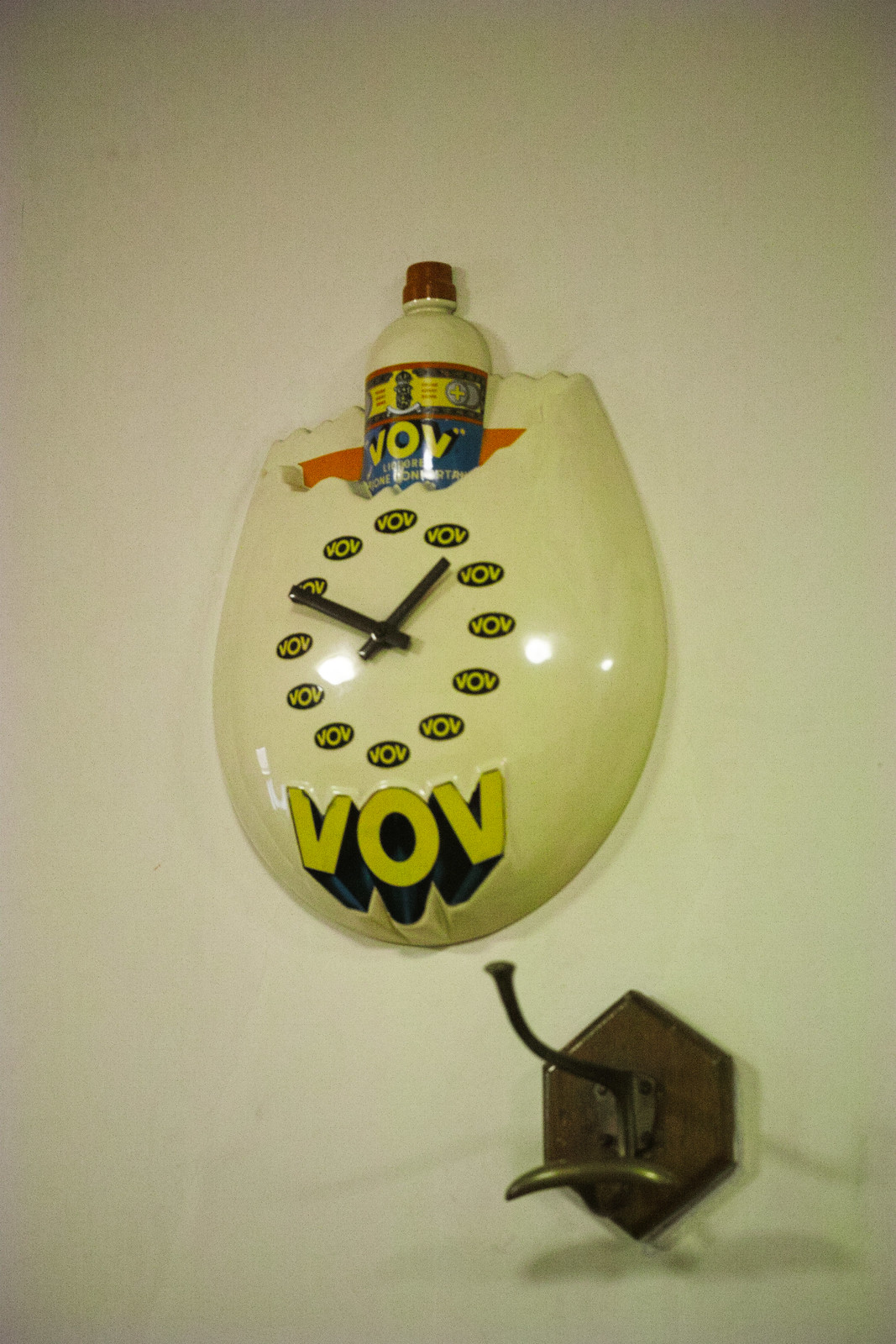The image depicts a large, egg-shaped, white wall clock that appears to double as a vintage advertisement for a product named "VOV." This intriguing clock features a bottle emerging from the top, resembling a bottle of liquor or soda with a blue label prominently displaying the name "VOV." Instead of traditional numbers, the clock face is uniquely marked with the word "VOV" in yellow lettering surrounded by black ovals at each hour, emphasizing the brand name. The clock, which seems to have a ceramic or plastic finish, is mounted on a completely white wall. Below the clock is a wooden coat hanger with metal hooks shaped in a hexagon pattern. This adds a functional yet aesthetic element to the setting, making the scene look perpetually like it’s always "VOV o'clock."